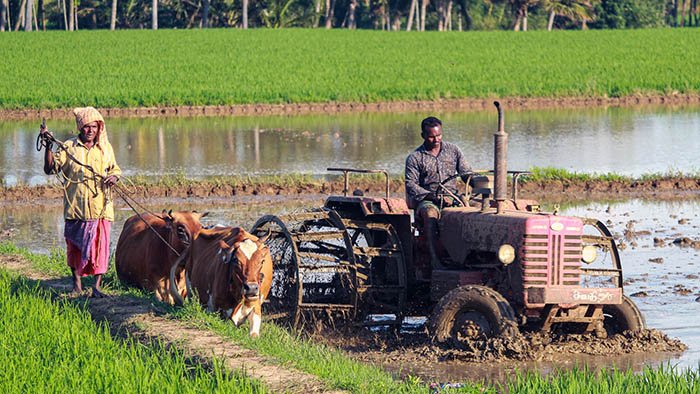The photograph captures a scene of farm life, possibly in a foreign country. At the very center of the image, a mud-covered red tractor is deeply stuck, and a man, seemingly trying to address the situation, sits atop the vehicle looking down. This man has an additional piece of fabric over his head, which complements his yellow button-up shirt and a sarong-like skirt in pink and purple hues. The tractor also appears to have a till attachment at the back, partially obscured by a group of light brown cows. To the left, another individual, a woman dressed in a yellow shirt, red skirt, and a head-covering shawl, is leading the cows using a brown rope. 

The cows, which have horns, are moving together along a tall, grassy area while the woman stands on an elevated path beside them. The background unfolds with a tranquil scene—a small river or lake reflecting the sunlight and the row of trees beyond. Beyond this body of water lies a vibrant, bright green, grassy field and the cropped trunks of about twelve trees reaching the top edge of the image. The overall setting suggests a moment of daily agricultural toil, captured amidst the serene but challenging beauty of rural life.